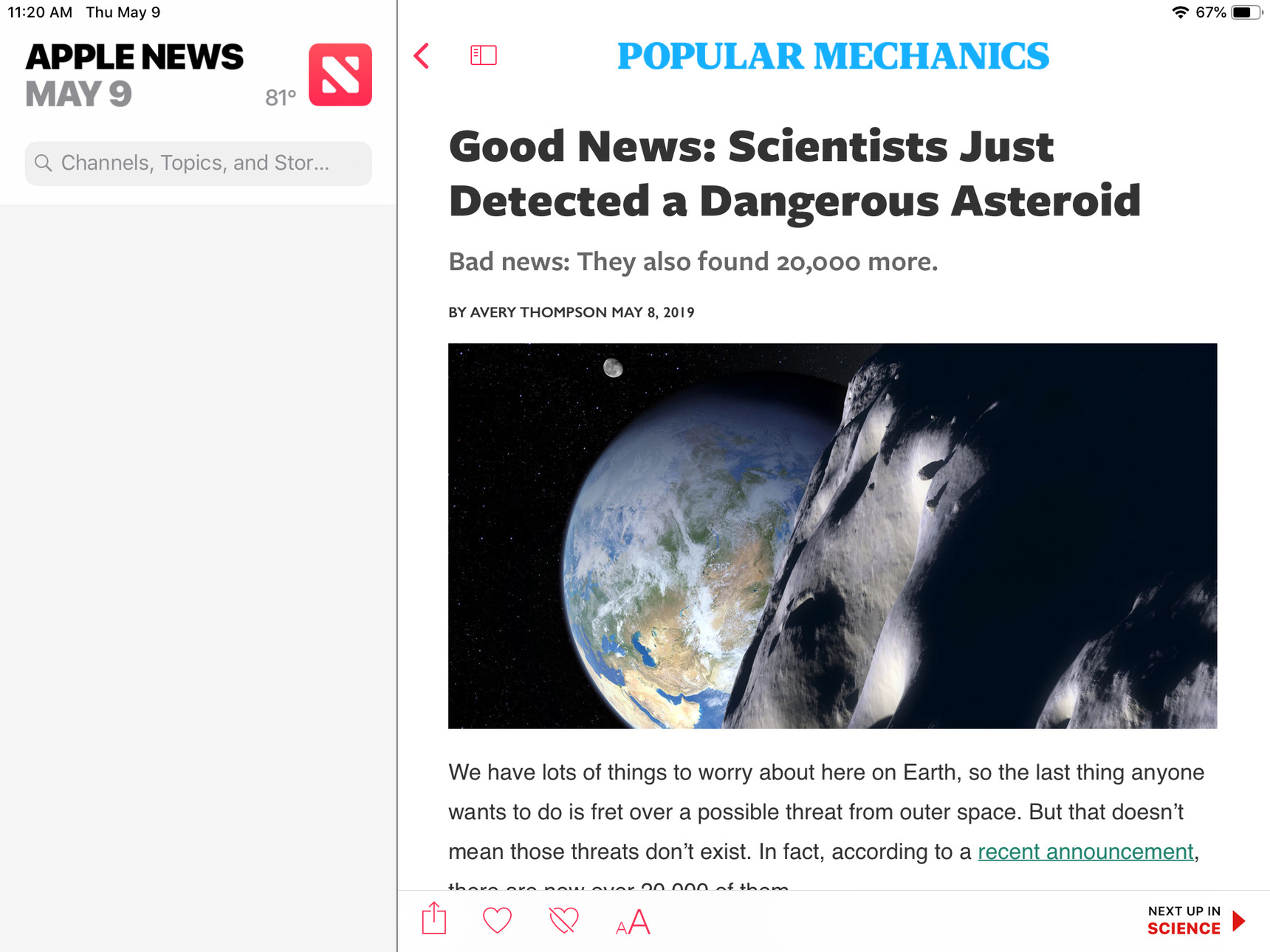The image appears to be a screenshot from a news reporting site, set against a white background. In the top left corner, "11:20 A.M." is prominently displayed in a distinguished dark gray font. Directly beneath it, the day of the week is abbreviated as "THU," followed by the date "May 9" in the same dark gray font. Below this, the words "APPLE NEWS" are written in bold, black, all-capital letters. Underneath "APPLE NEWS," the date "May 9" is repeated in gray, all-capital letters.

Approximately an inch to the right of this information, the temperature "81 degrees" is noted in gray font. Below this, there's an orange box with rounded edges, containing what appears to be a white letter, possibly an "N" or "S."

Directly beneath this setup, there's a light gray search box identifiable by a magnifying glass icon, suggesting it allows users to search by channels, topics, or stories, though the word "STORIES" is truncated to "STOR."

Further down, there's a large gray block, which might be a placeholder for additional content or imagery.

To the right side of the image, an article header is visible, featuring "POPULAR MECHANICS" in all-caps blue font. Just below it appears to be the title of an article: "Good News: Scientists Just Detected a Dangerous Asteroid."